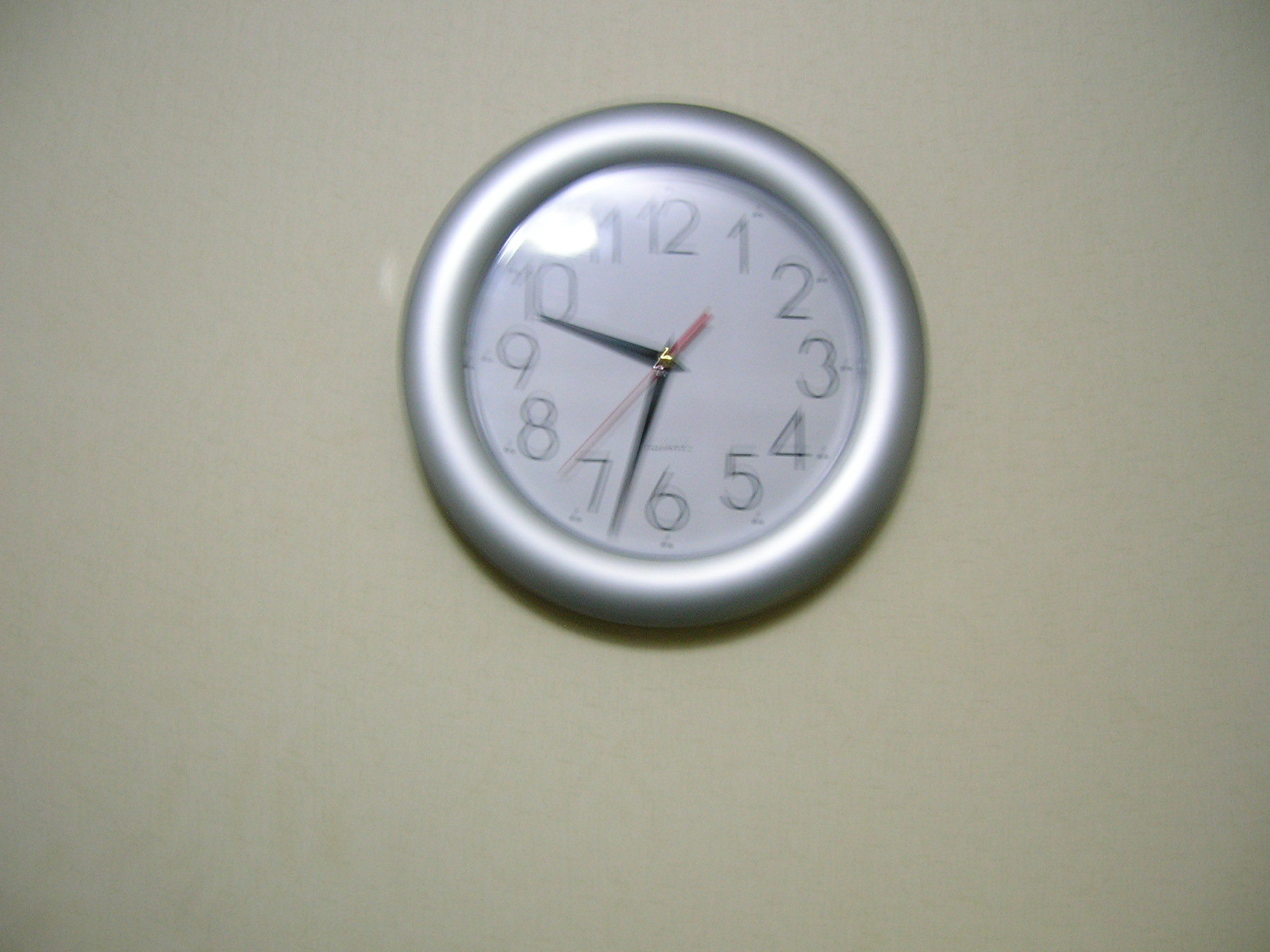This photograph features a wall-mounted clock with a prominent thick, rounded silver rim, set against a wall that appears almost grey in color, though it has been described as cream or light grey. The clock face is crisp white with bold, black numbers and corresponding black dots for each hour. The hour hand is a dark black, pointing close to 10, and the minute hand, also black, rests between 6 and 7. The clock features a thin red second hand situated between 7 and 8, with a slight golden reflection at its axis, likely from the central nut. Notably, there is some blurring in the image, possibly due to a flash reflection which creates an overexposed spot observed between the numbers 10 and 11. There is also an unreadable brand name just above the number 6 on the clock face.